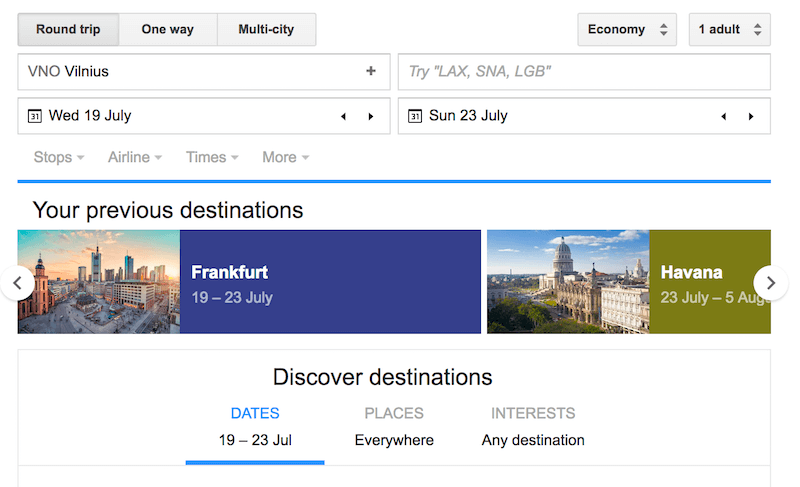A user is navigating a travel search interface in this screenshot. At the top, there are options for "Roundtrip," "One-way," and "Multi-city," with "Roundtrip" currently selected. The search specifications include "Economy," "One Adult," with the departure from "Vienna", and the destinations listed as "Vilnius," "Tri-LAX," "SNA," and "LGB." The travel dates are set from "Wednesday, 19 July" to "Sunday, 23 July." Additional filtering options listed are "Stops," "Airline," "Times," and "More."

The image also references previous search destinations such as "Frankfurt" (with travel dates from "19 through 23 July") accompanied by a photograph of the Frankfurt city skyline, and "Havana" (with dates from "23 July to 5 August") alongside a photograph of the Havana, Cuba skyline.

Further down, the interface displays "Discovered Destinations" with customizable parameters such as "Dates: 19 through 23 July," "Places: Everywhere," and "Interests: Any Destination." A blue horizontal line runs underneath these headers for emphasis.

The screenshot is purely illustrative and contains no people, animals, birds, mountains, automobiles, motorcycles, bicycles, or airplanes.